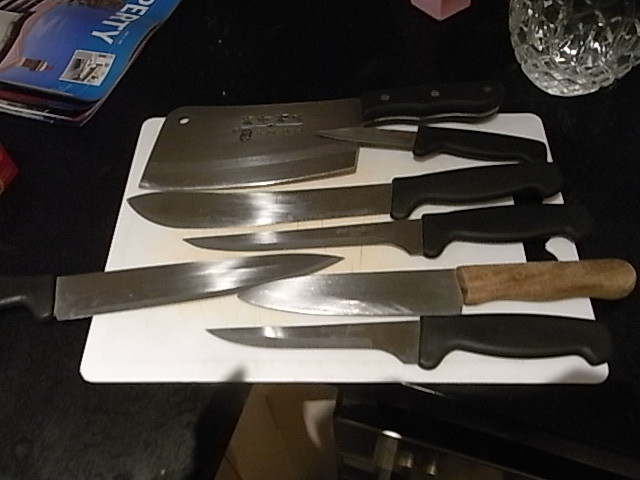A collection of seven kitchen knives, including a cleaver, is neatly arranged on a white plastic cutting board with rounded edges, situated on the corner of a black kitchen countertop. The cutting board shows visible etches from previous use. Most of the knives have black handles, with the cleaver distinguishable by its three silver rivets, suggesting higher quality. The cleaver's blade also bears some writing, possibly Japanese characters. Among the knives, there is one smaller paring knife, a butcher's knife, a fillet knife, and two all-purpose knives — one with a wooden handle and the rest with black handles. Notably, one knife's handle points left, contrasting with the others' right-hand orientation.

In the upper left corner of the image, there is a blue magazine titled "Liberty," though the first few letters are cut off. The cover features a rooftop and sky, with an indecipherable black and white square. In the upper right, there is a bumpy glass vase, alongside a pink rectangular object. Below the countertop, a dishwasher’s top edge is faintly visible, and the walls underneath appear light-colored, shadowed by the overhanging counter. The overall setting conveys a sense of organized but casual kitchen activity.